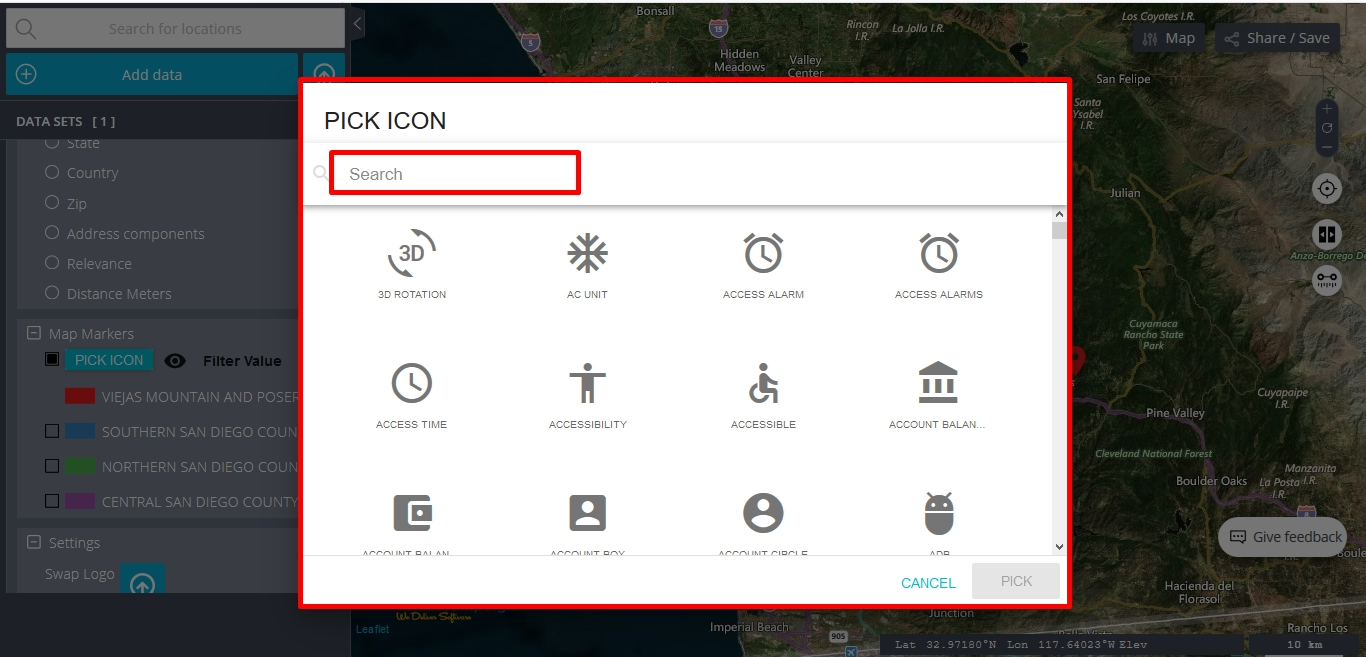The image is a rectangular screenshot with its longer side extending horizontally from left to right. The main focus of the image is a pop-up window centered within a grayed-out background. The pop-up window is outlined in red and features a white background.

At the top left corner of the pop-up window, the text "Pick Icon" is displayed. Just below this, there is a search box with the placeholder text "Search Unit," also outlined in red.

A horizontal gray line divides the window, and below this line, a set of icons is presented.

1. The first icon is labeled "3D Rotation" and depicts arrows rotating around a circle indicating a 3D transformation.
2. The second icon represents an air conditioning unit with the label "AC Unit."
3. The third icon is a simple alarm clock with the label "Access Alarm."
4. The fourth icon is another alarm clock labeled "Access Alarms."
5. The fifth icon displays a clock face with the label "Access Time."
6. The sixth icon features a figure with arms outstretched and is labeled "Accessibility."
7. The seventh icon shows a person in a wheelchair and is labeled "Accessible."
8. The eighth icon resembles a traditional bank, representing "Account Balance."
9. The final icon is a gray square overlaid with another smaller square, though the text label for this icon is unreadable.

This detailed description encapsulates the layout and contents of the image, providing clear information about each element within the pop-up window.